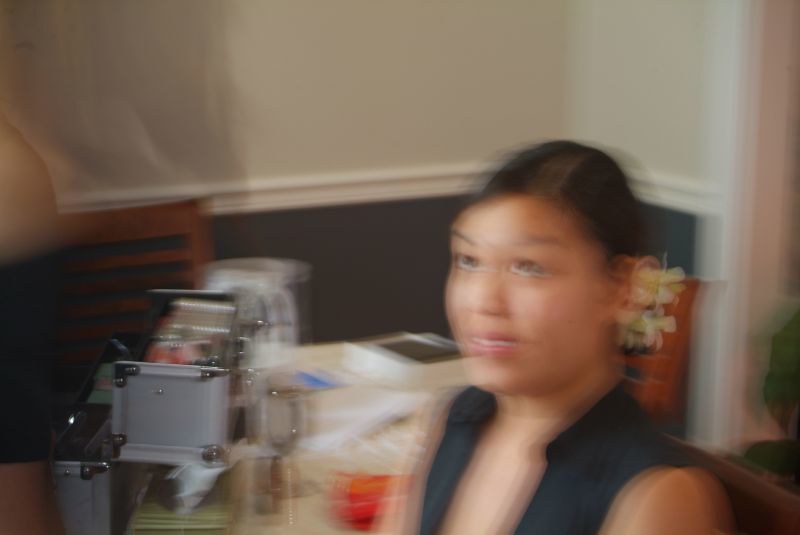The image is a blurred photograph of a dark- or tan-skinned woman sitting at a restaurant table. She is wearing a sleeveless, black, low-cut top, and has dark hair that may be neatly pulled back or parted in the middle, with a flower adorning her hair. The focus is around her chest up, making finer details unclear due to the blurriness. The background features a table with various indistinguishable items piled on it, including something that appears to be a container. Behind the table, there is a wall separated by dark-brown paneling at the bottom and an off-white color above, with a white doorframe trim visible on the right edge of the image.